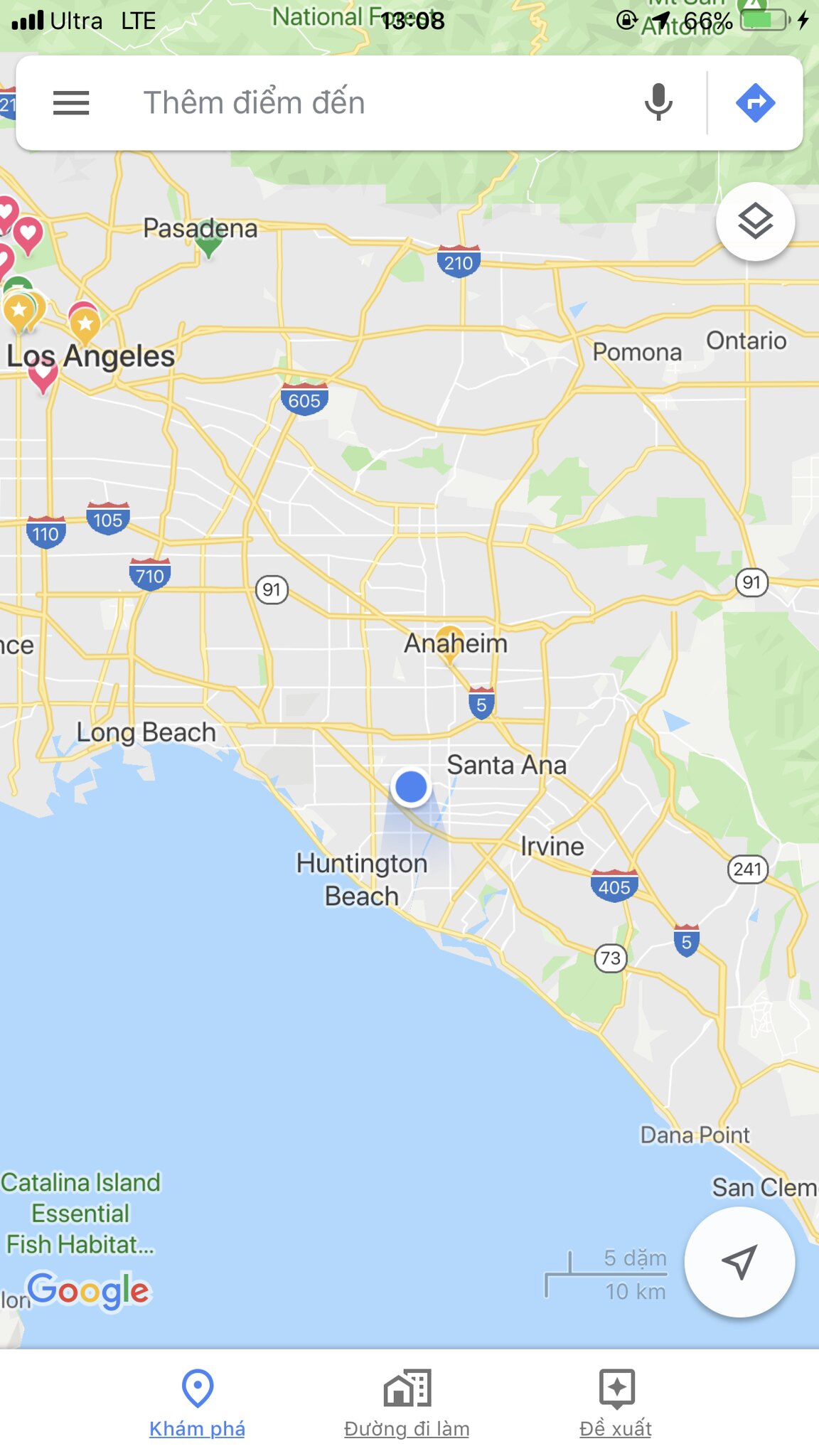The image features a close-up of a Google Maps screenshot displayed on a smartphone, centered on Southern California. The map prominently showcases the region between Los Angeles and San Diego. In the upper left-hand corner, Los Angeles is clearly visible. The display follows the course of Interstate 5, highlighting key cities including Anaheim, Santa Ana, and Irvine, with Huntington Beach and Long Beach marking coastal landmarks. To the north, the cities of Pomona, Ontario, and Pasadena are also noted.